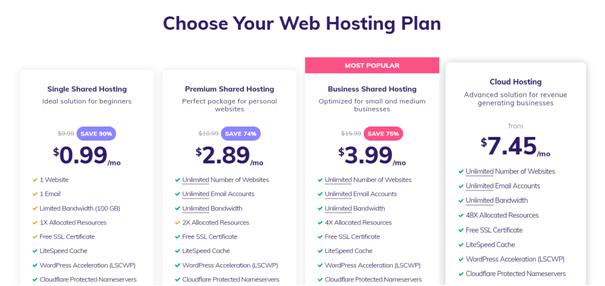The image displays a selection of four web hosting plans under the heading "Choose Your Web Hosting Plan." 

1. **Single Shared Hosting**:
   - **Description**: Ideal solution for beginners.
   - **Discount**: Save 90%.
   - **Price**: $0.99 per month.
   - **Features**: Lists the various features and options included in this plan.

2. **Premium Shared Hosting**:
   - **Description**: Perfect package for personal websites.
   - **Discount**: Save 74%.
   - **Price**: $2.89 per month.
   - **Features**: Detailed features and options provided with this plan.

3. **Business Shared Hosting**:
   - **Highlight**: Marked as the "Most Popular" option with a pink banner.
   - **Description**: Optimized for small and medium businesses.
   - **Discount**: Save 75%.
   - **Price**: $3.99 per month.
   - **Features**: Comprehensive list of features and options included with this plan.

4. **Cloud Hosting**:
   - **Description**: Advanced solution for revenue-generating businesses.
   - **Price**: Starting from $7.45 per month.
   - **Features**: Includes unlimited number of websites, unlimited email accounts, unlimited bandwidth, a free SSL certificate, and LiteSpeed Cache, among other features. 

Each plan summarizes the advantages, pricing, and specific features to help users make an informed decision about their web hosting needs.